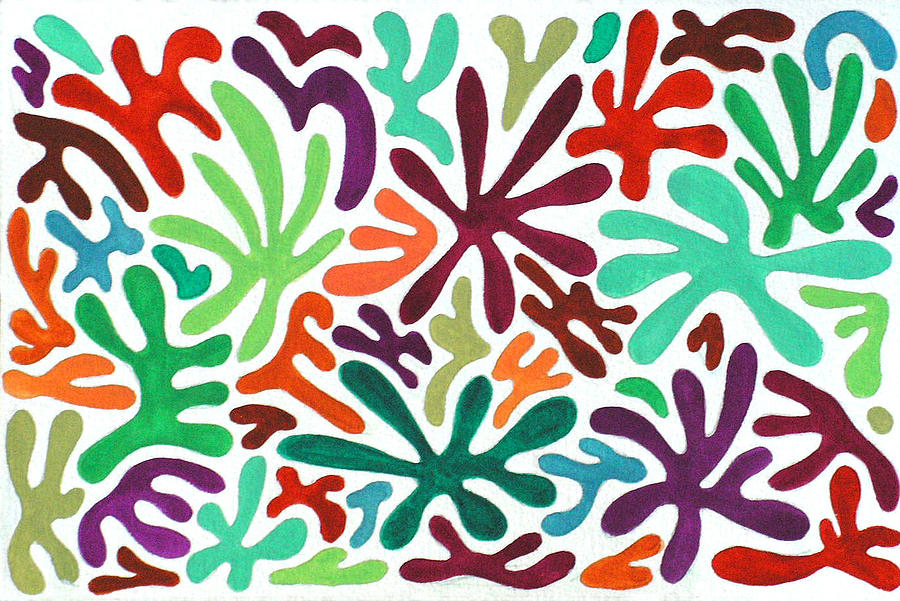This artwork is an abstract painting, possibly created using markers or watercolor, characterized by its vibrant and intricate design. The piece features an array of interconnected shapes, reminiscent of undersea coral or wildflowers, with each shape having spindly legs extending from it. These shapes come in a variety of colors including reds, blues, purples, maroons, oranges, lime greens, avocado greens, browns, and burgundy. The artist has meticulously arranged these shapes to fit together loosely, minimizing white space while ensuring that no two colors are exactly the same. This creates a refined and almost patterned appearance on the white background, filling the entire canvas with a dynamic and engaging composition. The piece exudes a sense of harmony and randomness simultaneously, akin to what one might find in a modern art museum.